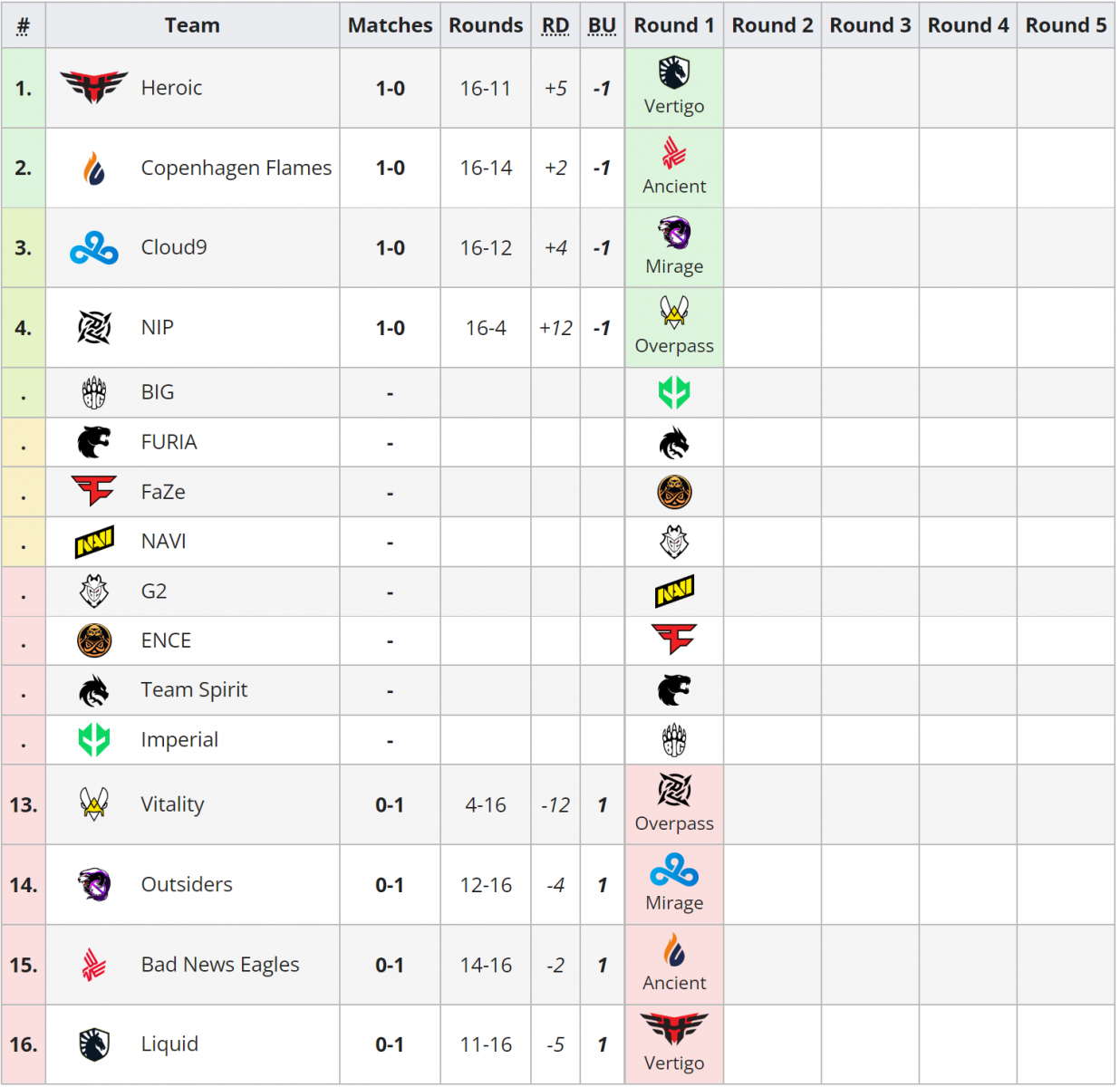A detailed spreadsheet is displayed, featuring a comprehensive overview of various sports teams' performances. The spreadsheet consists of 17 rows (including the header) and 11 columns. The columns are labeled as follows: "Number" (1 through 16), "Teams," "Matches," "Rounds," "RD," "BU," and rounds 1 through 5. 

The first two rows are highlighted in light green, indicating the top-performing teams. The teams Heroic and Copenhagen Flames are listed here, with match records of 1-0 each. Heroic's scores are detailed as 16-11, and 16-14 for Copenhagen Flames. The spreadsheet also indicates which teams they defeated in round 1.

Conversely, at the bottom, rows 15 and 16 feature Bad News Eagles and Liquid, who have losing records. Additionally, the spreadsheet includes the logos of all the teams, providing a visual reference for each. This detailed layout offers a clear and organized view of the teams' current standings, match results, and round performances.